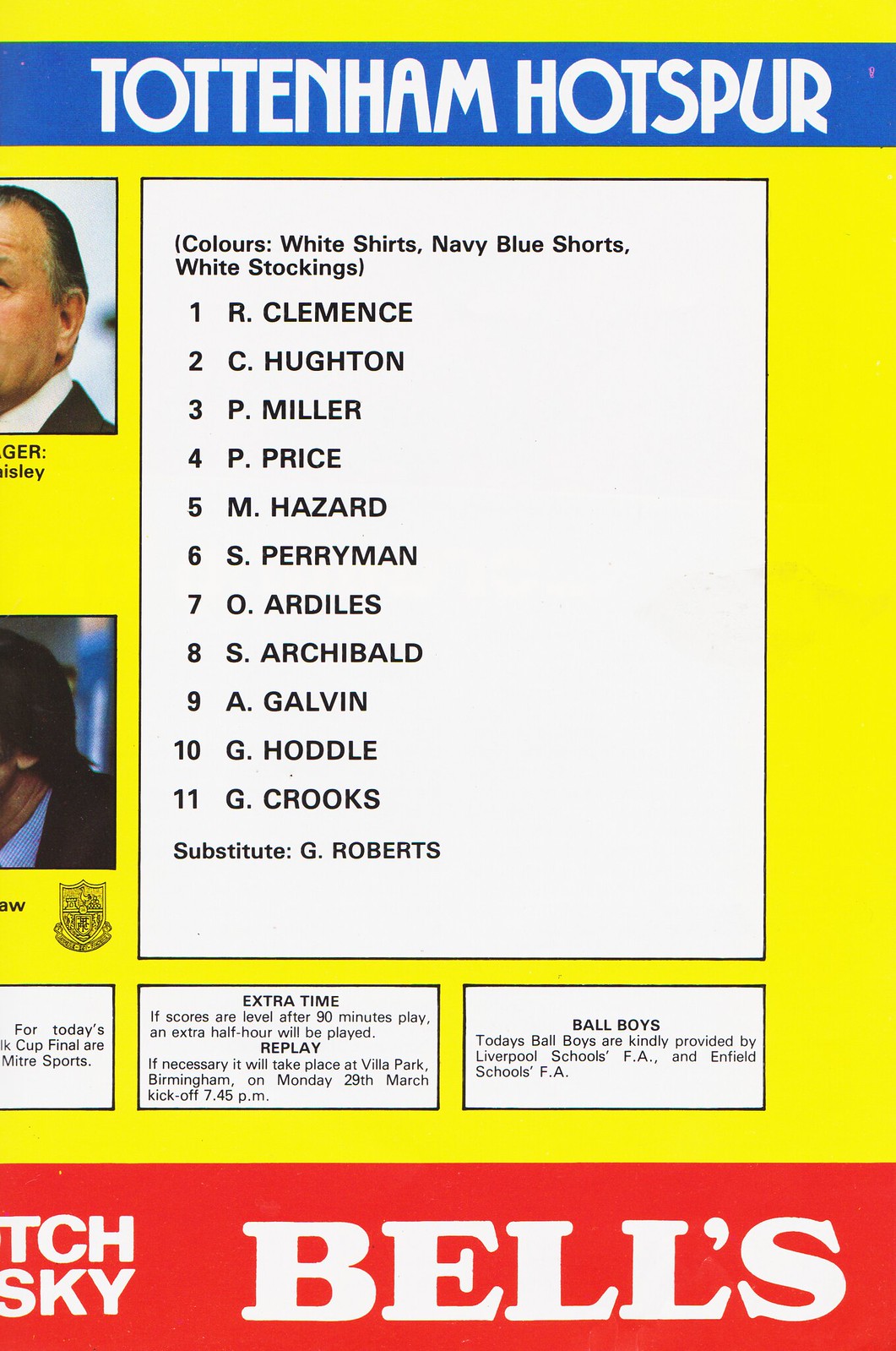The image is a photograph or scan of a page that appears to be part of a book or advertisement, distinguished by its vibrant yellow background. At the very top, a blue banner stretches across the image bearing the words "TOTTENHAM HOTSPUR" in bold, capitalized white letters. Centered in the middle of the image is a large white box containing black text. This text outlines the team colors as "white shirts, navy blue shorts, white stockings" and lists the team roster numbered from 1 to 11: R. Clements, C. Hewton, P. Miller, P. Price, M. Hazard, S. Perryman, O. Ardiles, S. Archibald, A. Galvin, G. Hoddle, and G. Crooks, along with substitute G. Roberts.

Below this roster box are two smaller white boxes aligned in a row. The left box discusses extra time and replay information, stating, "If the scores are level after 90 minutes play, an extra half hour will be played. Replay if necessary will take place at Villa Park, Birmingham on Monday 29th March kickoff 7:45 p.m." The right box is labeled "Ball Boys."

The bottom edge of the image features a red banner with the word "BELLS" in white capital letters. There is additional text along the left and parts of the image that are cut off or unreadable. Also present on the left side are portions of two color photographs of men's faces, although these are largely obscured by the edge of the image. The various colors in the image include red, white, yellow, blue, black, and gray.